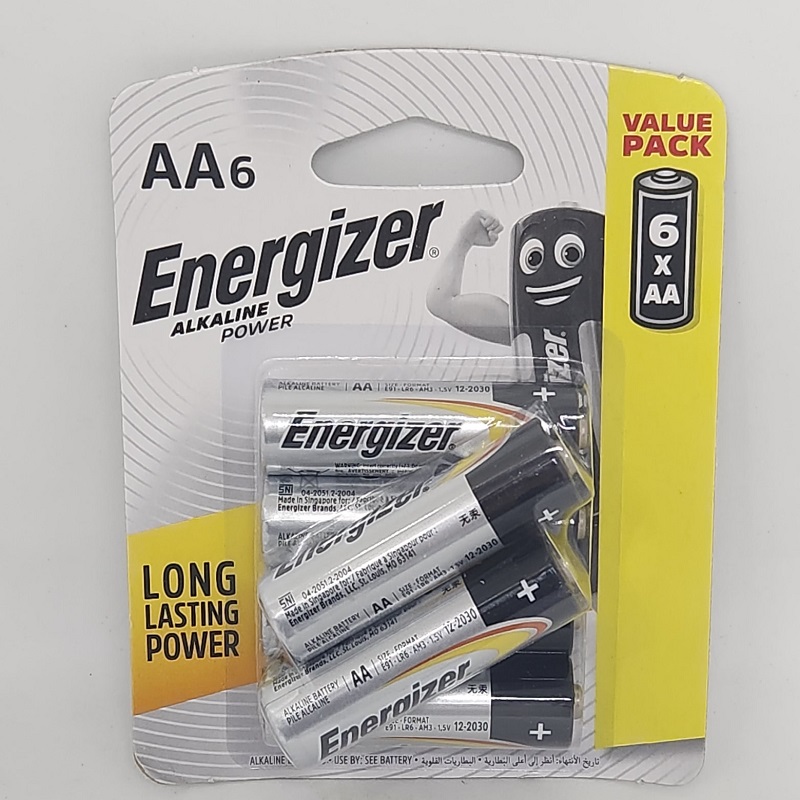The image is a close-up, vertically oriented photograph of an Energizer alkaline batteries product package. The background is a soft, light gray that accentuates the details of the packaging. The packaging consists of a cardboard backing and a clear plastic front, which displays the batteries inside.

Prominently featured on the right side of the cardboard backing is a vertical yellow banner with the words "Value Pack" written in bold red letters at the top. Directly beneath this banner is an image of a battery labeled "6 x AA," indicating the quantity of AA batteries contained in the package. Just left of the yellow banner, a battery character is depicted with bright eyes and a wide smile. The character's right arm is extended and flexed upwards at a 90-degree angle, showcasing a strong bicep.

Enclosed within the clear plastic front are six AA batteries. Four of these batteries are aligned vertically, one above the other. The remaining two batteries are positioned diagonally over the top four, running from the lower left to the upper right. This arrangement not only emphasizes the quantity but also adds a dynamic visual element to the packaging.